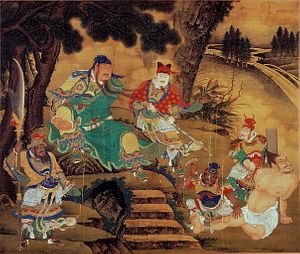This is a detailed depiction of a historical Chinese painting or illustration. The scene features a diverse group of individuals, with their costumes varying significantly. They are seated outdoors beneath two large trees, seemingly engaged in a gathering or possibly a picnic. Prominent among them is an individual in an ornate green robe adorned with gold, who could be an emperor or a noble, sitting with long hair or a Fu Manchu-style beard. This figure also wears a blue silk cap. Another notable character beside him is dressed in a red robe with gold designs and a gold silk cap, complemented by white kabuki face makeup. 

In front of these two figures is what appears to be a military guard, clad in a yellow-gold jacket over a white robe, holding a spear with a curved metal blade. Additionally, there's a figure in the lower right corner, minimally dressed in a white diaper-like garment. 

The background features a staircase with an off perspective, leading to a scene of dark green-leaved trees, a road through a forest, and a sunset in the upper right. The overall background color is predominantly yellowish-brown, adding a muted yet warm tone to the intricate scene. The painting may include a blend of humans and possibly deities, given the historical and mythical elements depicted.